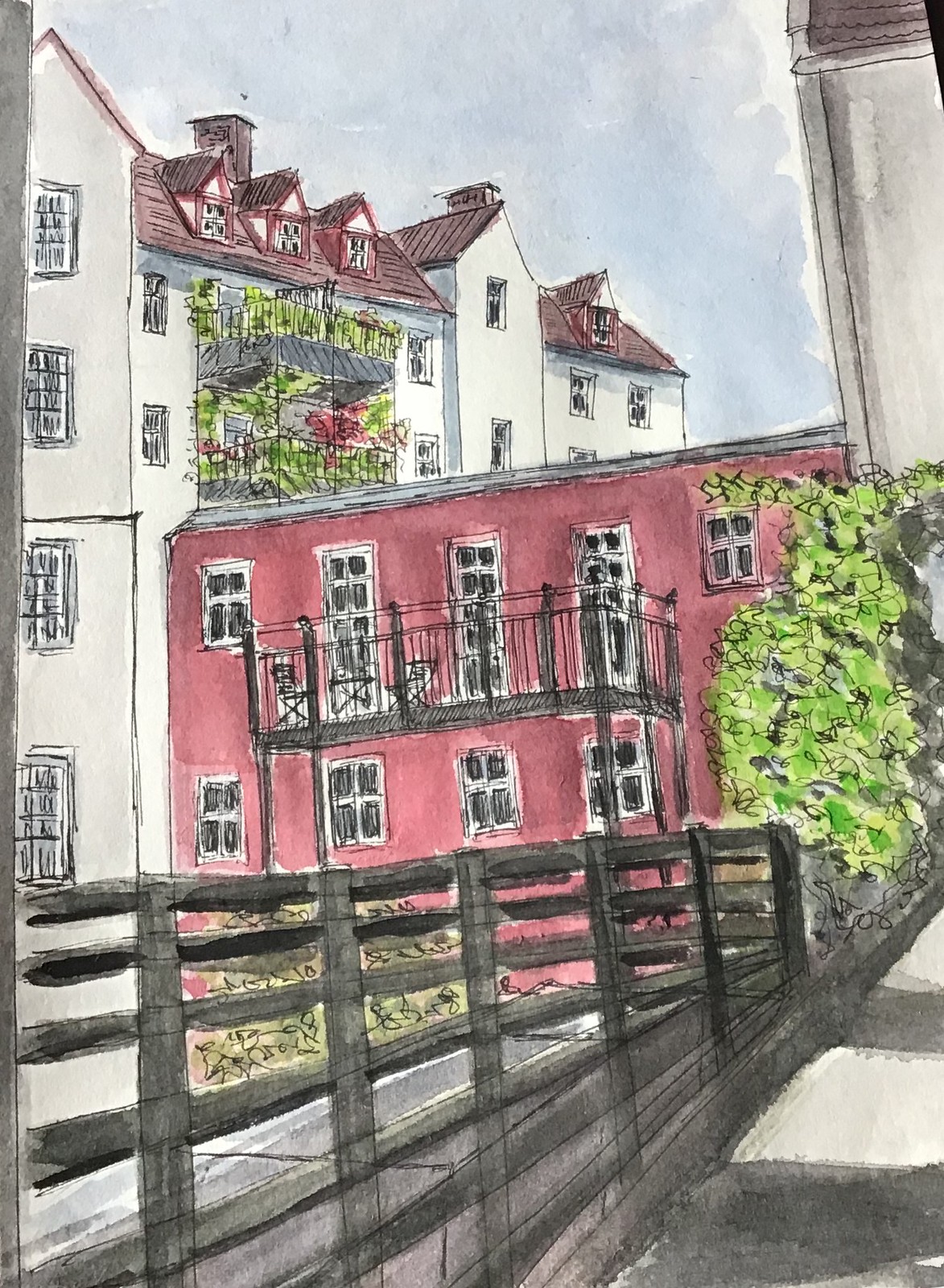The hand-drawn illustration, accentuated with watercolours, is presented in portrait orientation and depicts a scene of several buildings with intricate details. The foreground presents a walkway made of white stone interspersed with dark, muddy puddles, and a wooden railing painted in varying shades of brown runs along the left side in front of a thick stone wall. To the left, there’s a lower, maroon-painted building with horizontal, black, and white-framed windows and a grey roof. Adjacent to this building, on its rooftop, are planted trees with green foliage.

Dominating the background, a taller white apartment block stretches across the scene, featuring metal balconies adorned with plants in shades of green and red. This building also displays various dormer windows along its brown roofline and several chimney stacks. To the right of the maroon building stands a smaller, greyish structure with a shrub or small tree immediately in front. The detailed interplay of colors and architectural elements create a vivid and engaging urban landscape.